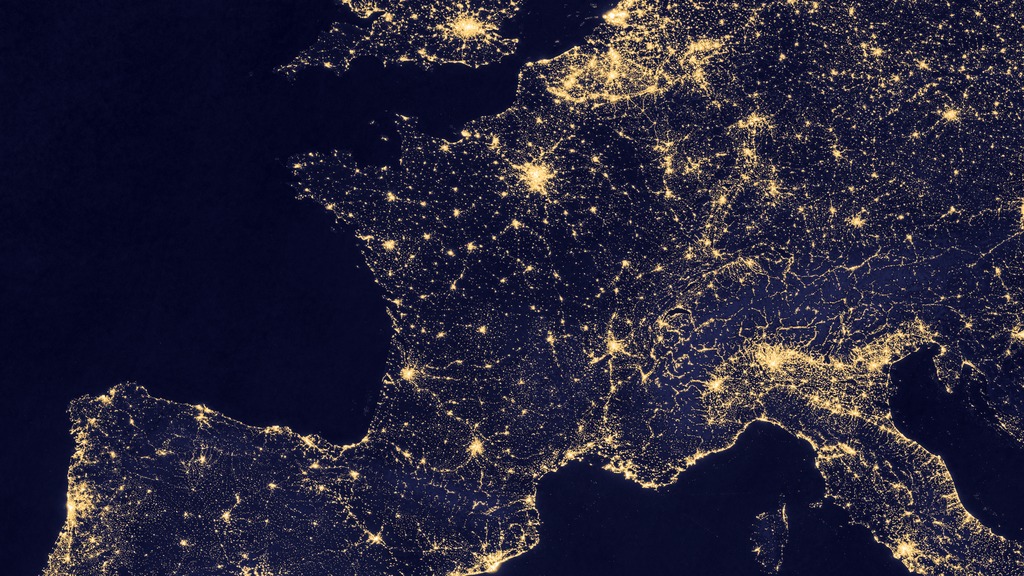This striking close-up image, taken by NASA, showcases an overhead nighttime view of parts of Earth, specifically highlighting southwestern Europe and Australia. Set against a deep black and navy-blue background, the image vividly captures the spatial distribution of human settlements through an array of bright, golden lights. These lights are scattered across various regions, depicting major cities and densely populated areas.

At the top of the image, a small piece of land can be seen, bathed in subtle hues of gold, resembling a star-studded night sky. Central to the image is a larger landmass, with luminous gold streaks and flashes marking prominent locations. The lower right corner features a distinctive, peninsular shape, also highlighted with sporadic patches of gold light. To its left, a small island is visible, similarly illuminated.

In this captivating image, each landmass is rendered in shades of dark to lighter blue, with the glittering gold lights creating the illusion of cracks and veins across the continents. This detailed visual not only emphasizes the sprawling extent of human civilization but also presents an ethereal, almost celestial perspective of our planet as seen from space.